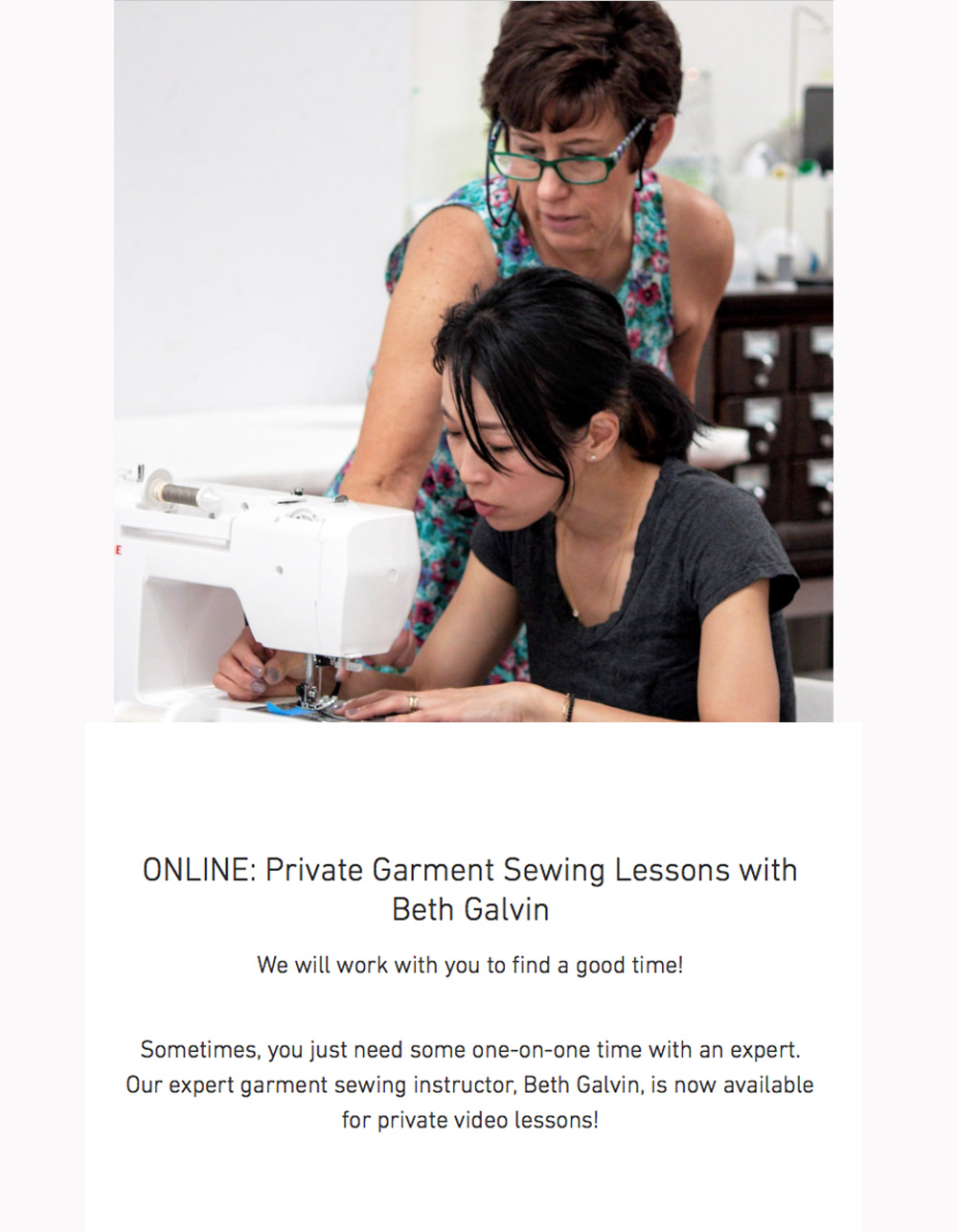In this promotional image, an older white woman with short brown hair, wearing glasses, and dressed in a turquoise blue summery dress adorned with pink and white flowers, is standing and leaning over a younger Asian woman. The younger woman, seated and focused on her task, is working at a white sewing machine. She is dressed in a short-sleeved black t-shirt with a low collar and silver stud earrings. The older woman, presumably Beth Galvin, is guiding or pointing out something on the sewing project. The image is part of an advertisement for "Online Private Garment Sewing Lessons with Beth Galvin," stating, "We will work with you to find a good time. Sometimes you just need some one-on-one time with an expert. Our expert garment sewing instructor, Beth Galvin, is now available for private video lessons." The photo sits above a white rectangle with black text and is bordered by light gray on the left and right sides.